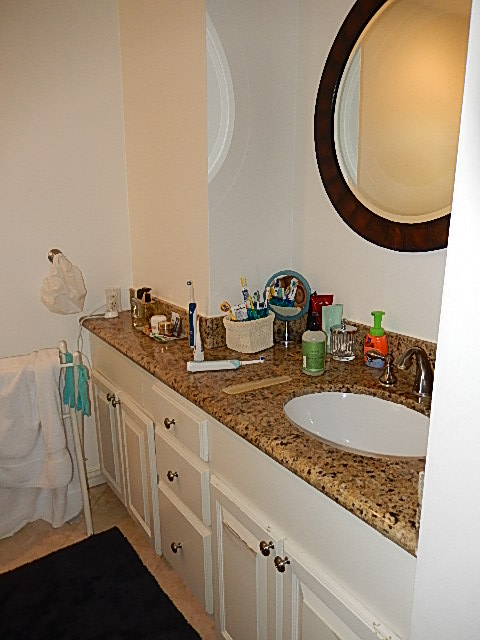The photograph captures a detailed scene in a bathroom taken in portrait mode. In the upper right-hand corner, a round oval mirror with a brown wooden border is prominently featured. The mirror reflects the wall behind it and a mysterious white curved paint mark on the left side. The upper left-hand corner transitions into a dark cream-colored wall, which indents and blends into a creamier-colored wall. This indentation and a potential light source are also visible in the mirror's reflection.

At the bottom left-hand corner, the dark cream tiled floor is partially covered by a black floor mat. Above the floor mat and towards the left center, a plastic towel holder in cream color holds a white towel, with two small green gloves hanging nearby. A wall hook carries a plastic hair cap. 

The bathroom counter, designed with a dark cream base and marbled with black and light cream accents, is cluttered with various toiletries for brushing teeth. An aqua-colored mirror, the sink, and cabinetry complete the depiction of this everyday, yet intricate bathroom setting.